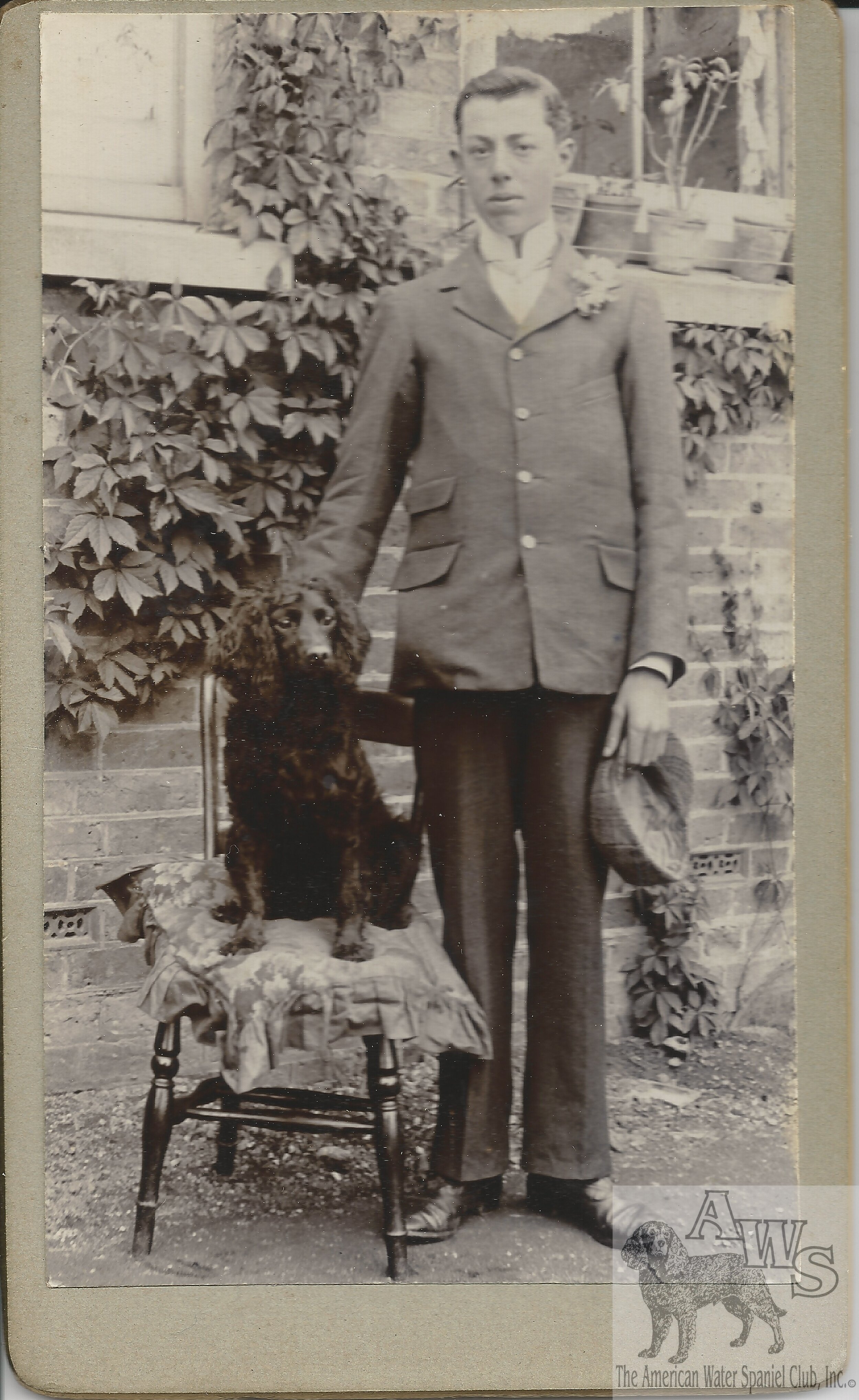This black and white, vintage photograph captures a young, Caucasian man standing next to his black, furry-coated dog, which is seated on a cushion-topped wooden chair. The man, dressed in formal attire consisting of a grey coat over a high-collared white shirt, dark pants, and black shoes, holds a plaid cap in his left hand while affectionately touching the dog. The background features a brick wall adorned with ivy and a prominent window, with several potted plants visible in the top right corner. The inset at the bottom right shows an illustration of a dog with the block letters 'AWS,' indicating the American Water Spaniel Club, Inc. The man looks directly at the camera with a composed expression, completing the nostalgic aura of the historical outdoor setting.